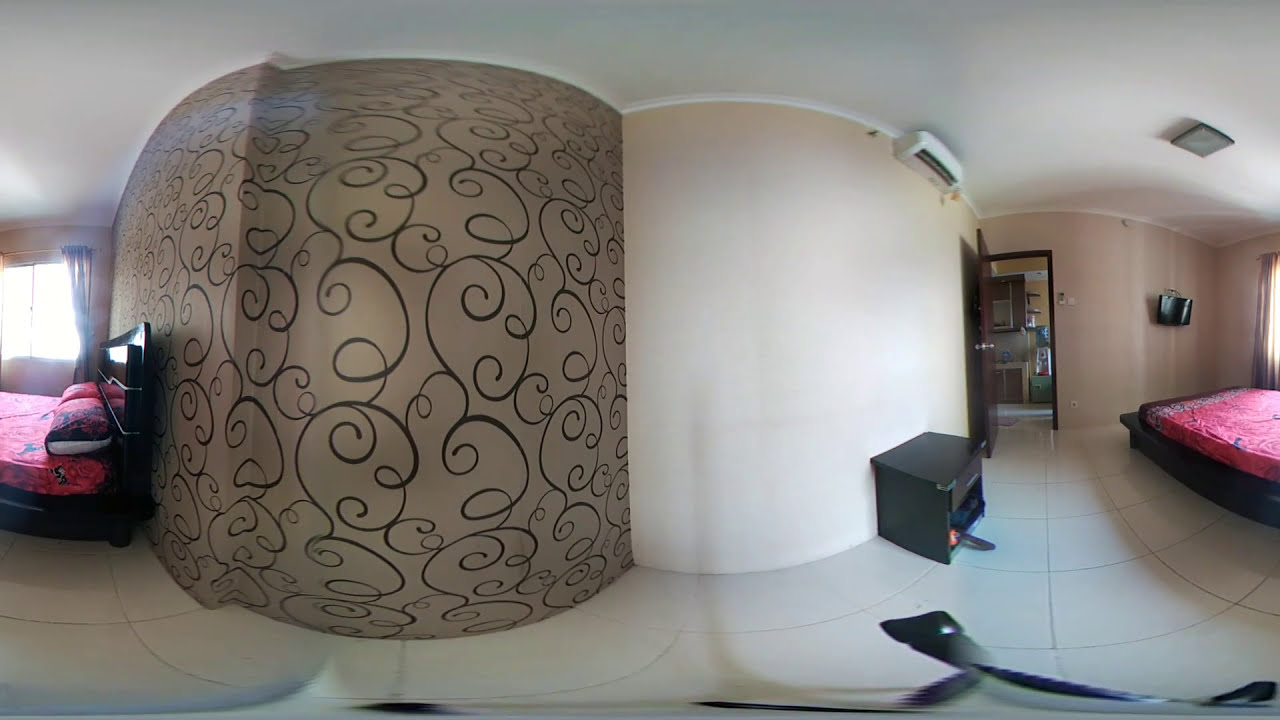The image is a 360-degree panoramic view of a bedroom with white tile flooring and a white ceiling. The bed, located centrally in the room, has a black frame with red sheets and pillow coverings. The wall behind the bed is adorned with dark brown and beige wallpaper featuring black swirls. Surrounding walls are a beige or cream color. Near the center of the right wall, there is a rectangular air conditioner mounted close to the ceiling.

To the right of the bed is a window with two glass panes, through which sunlight streams. Adjacent to the window, on the far right side, you can spot the edge of a curtain. Moving towards the left from the window, there's a small black nightstand. Further to the right, there's a doorway leading to what appears to be another room, possibly a kitchen, and on the wall beyond the doorway is a wall-mounted TV. Below the air conditioner, at the bottom right of the image, a small black chest or drawer is visible.